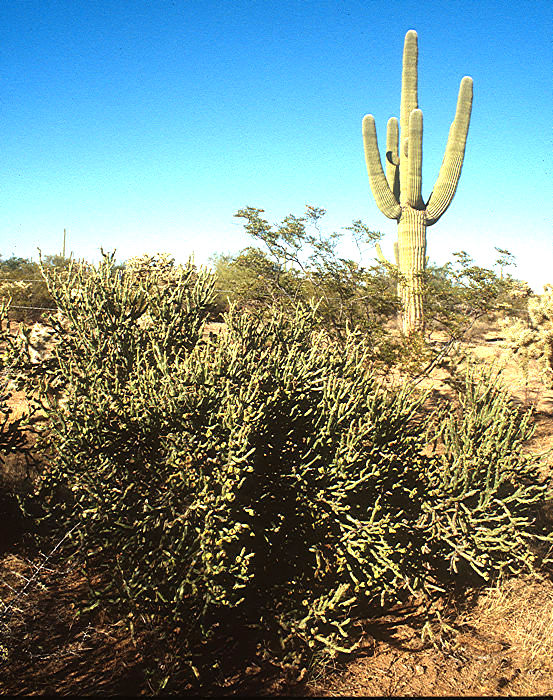This is an image of a desert landscape on a sunny day. Prominently featured in the background is a large cactus with five green stalks, getting wider toward the base. Surrounding and beneath the cactus are numerous light green bushes and shrubs, light green in color and resembling finger-like leaves, which are sturdy and a bit dried. The arid climate is evident from the dry, sandy, and whitish-tan ground, which looks parched and water-starved. The sky above is a striking, uninterrupted blue, devoid of any clouds. This scene encapsulates the essence of a typical desert environment with its clear sky and diverse arid vegetation.